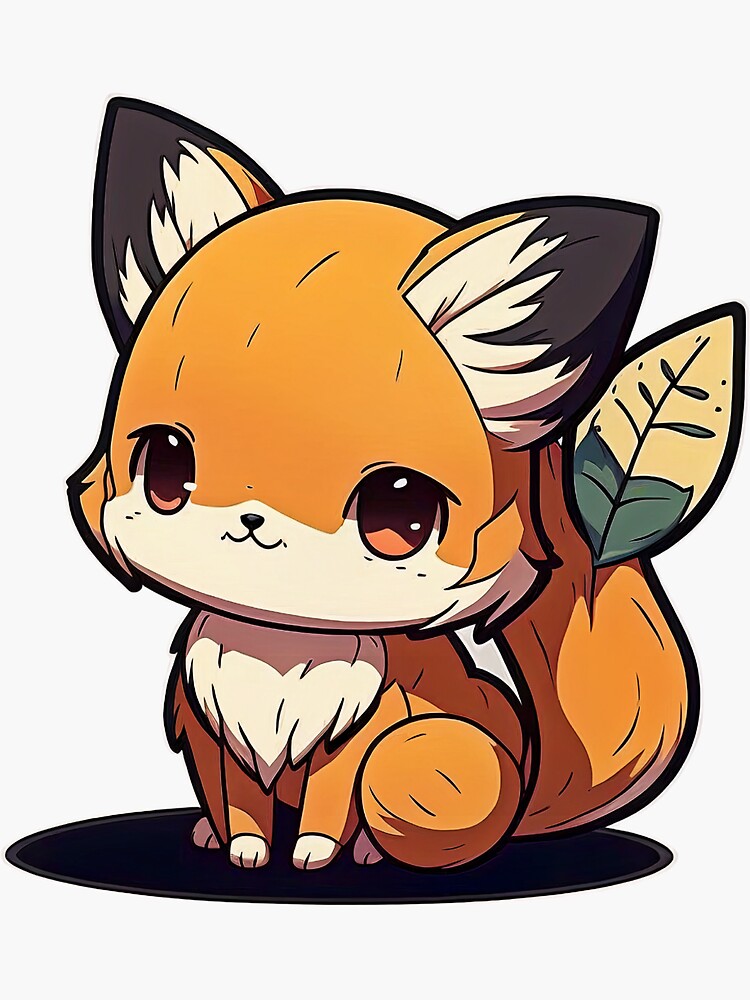The image showcases an anime-style cartoon fox with a predominantly orange body set against a white background. The fox, resembling the Pokémon Eevee, features large, pointed ears with black tips fading into a beige color. Its face, which is somewhat humanoid, exhibits large, exaggerated black eyes with orange and white highlights, small, cute black nose, and a tiny black mouth. The lower half of its face and the puff of fluffy fur on its chest are white. The fox's limbs have white paws, and it has a large, fluffy orange tail with a single leaf protruding from it. The leaf has a light yellow and green gradient. The character sits on a flat, black circular shadow which emphasizes the light coming from above, accentuating the detailed and charming design of this adorable fox-like figure.